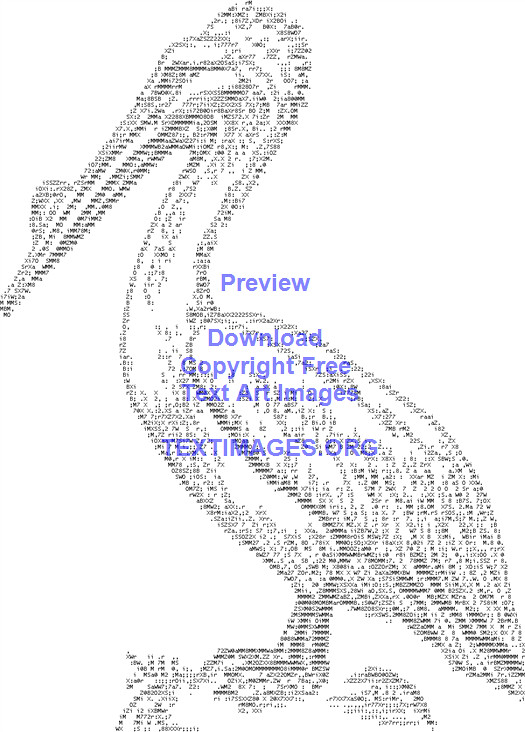The image displays a digitally-rendered pelican, meticulously crafted from a variety of keyboard symbols like N's, M's, O's, 7's, X's, and more, all against a pristine white background. The pelican, detailed enough to clearly depict its standing posture on what appears to be a small tuft of grass or a rock, is centrally positioned. A subtle yet visible thin diagonal line spans from the bottom left to the upper right and then across, adding a minimalist touch. Notably, there is an indistinguishable object, possibly a fish, in the bird's beak, indicating it is carrying something. Prominently, bold blue text overlays the center of the image, reading "PREVIEW, DOWNLOAD COPYRIGHT FREE TEXT ART IMAGES, TEXTIMAGES.ORG," suggesting the image is sourced from this website and a watermark-free version might be available for download. The color scheme prominently features black, white, and blue, embodying the digital art style characteristic of text art.